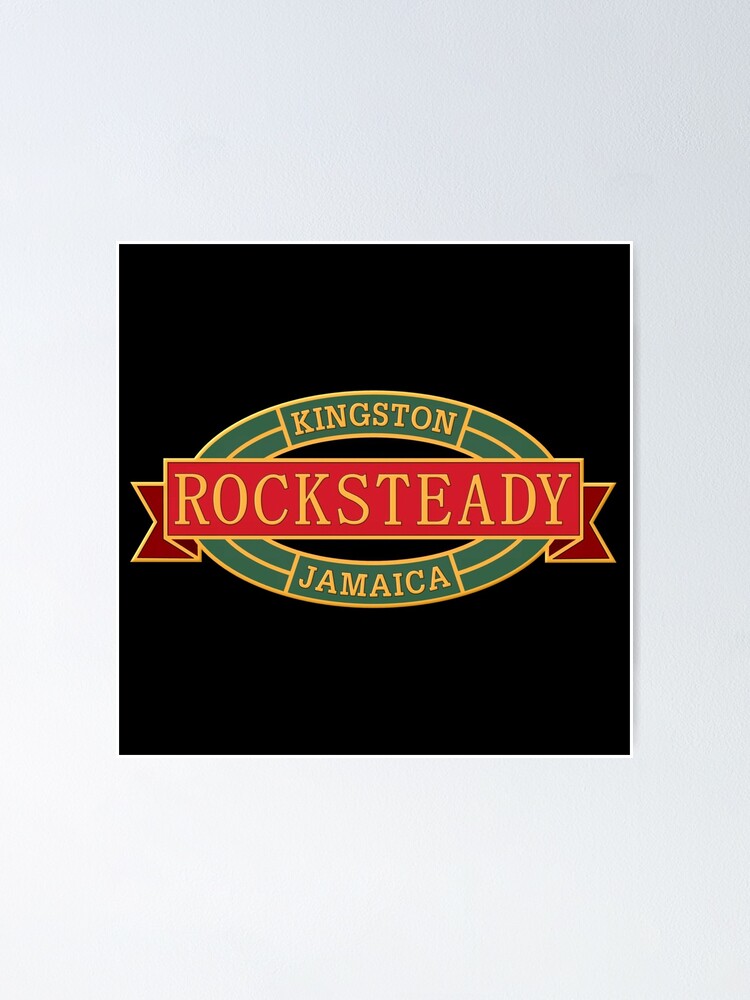The image displays a minimalist logo featuring the colors of the Jamaican flag: green, red, and yellow. Central to the design is a green circle set against a black backdrop. At the top of the circle, "Kingston" is written in yellow text, while "Jamaica" is written at the bottom. Dominating the center of the green circle is a bold red banner with the words "Rock Steady" in yellow lettering. The outer border of the circle is green, complementing the overall color scheme. The design employs simple, flat matte colors with straightforward, standard font choices, conveying a clean and uncluttered aesthetic. There are no additional images or text, focusing solely on representing Kingston, Jamaica, and the Rock Steady genre in a stylized yet understated manner.